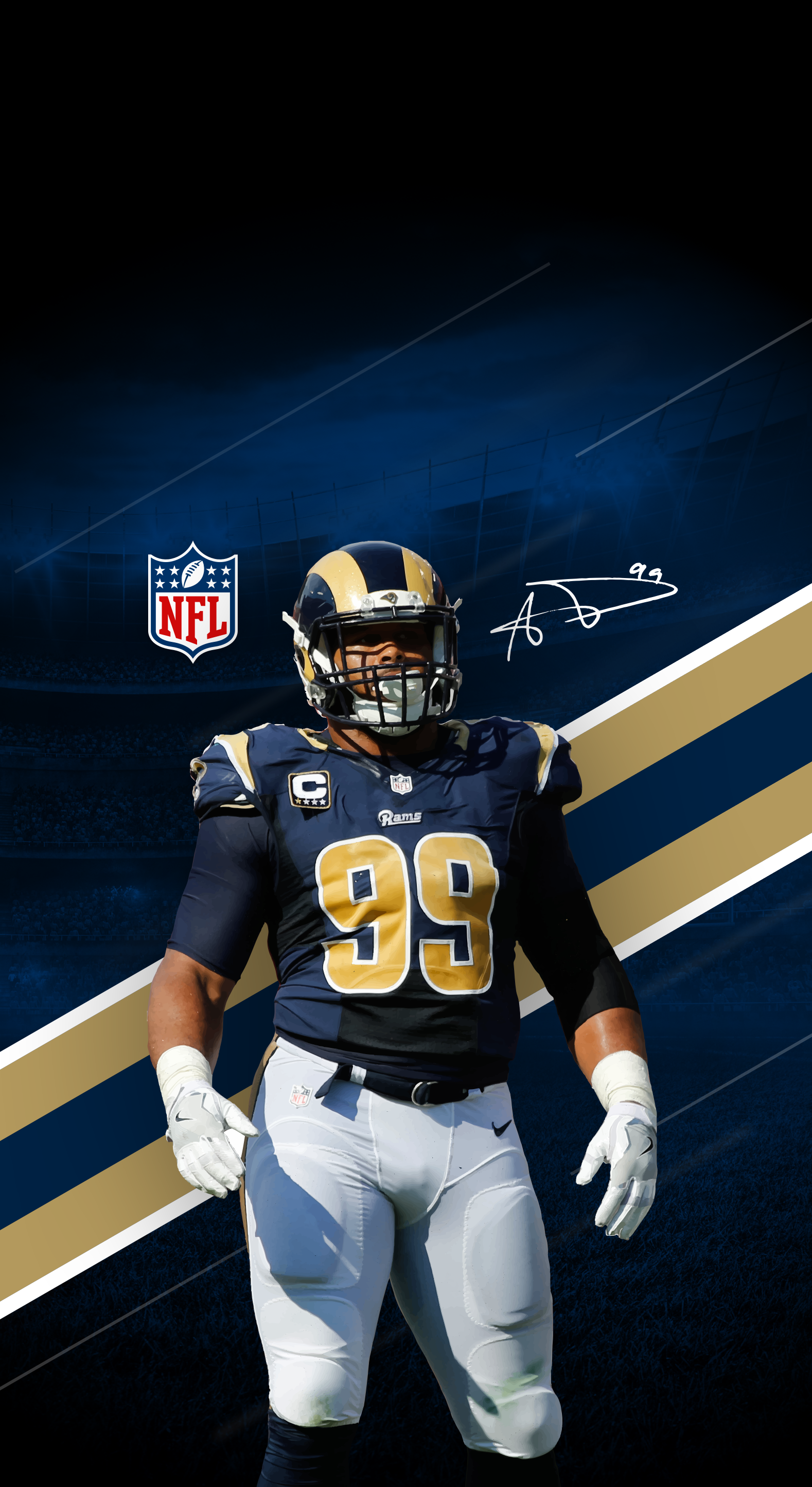The image depicts Aaron Donald in his St. Louis Rams uniform, characterized by a dark navy blue jersey with gold numbers and accents. He sports the number 99 prominently on his chest, with "Rams" inscribed above it and a captain's "C" patch on his left shoulder, bordered in gold with stars underneath. Donald's attire includes white pants with padded thighs and knees, a blue belt, and white Nike gloves. His wrists are taped with white athletic tape, and he wears a tight, dark blue undershirt beneath his jersey.

His helmet is navy blue, decorated with iconic gold ram horns. The NFL logo in red, white, and blue is visible over his right shoulder. Aaron stands in a neutral stance, not mid-play, against a backdrop featuring stripes in Rams colors and a faint rendering of a stadium with a gradient from black at the top to turquoise at knee level, turning black again near the bottom. His signature, "AD99," is positioned to the right, contributing to the overall impact of the image. This photograph captures Donald during the St. Louis Rams era, showcasing the bold and distinctive team colors and design elements.